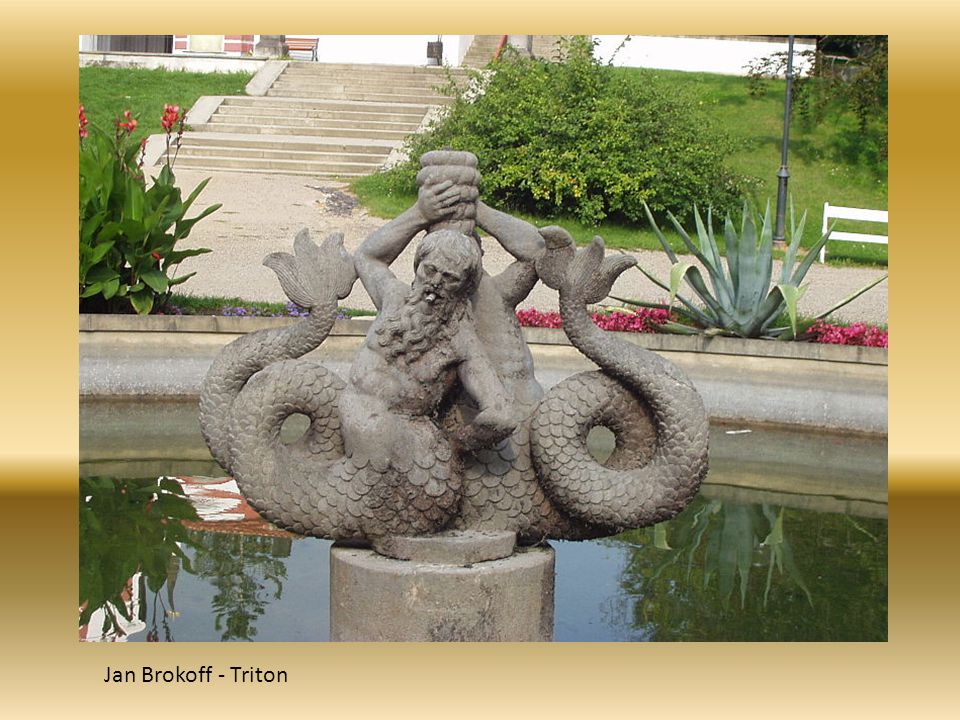The image depicts an intricately detailed concrete statue of two merpeople, each with a human upper torso and a fishtail. One merman, bearded, faces forward, while the other’s face is obscured as they both hold a vase above their heads, designed to spray water when the fountain is active. The statue sits on a pedestal within a greenish, somewhat murky water fountain that is encased by a concrete wall. Surrounding the fountain are various forms of vegetation including pink and purple flowers, ferns, bushes, and grass. The scene appears to be situated in a garden or possibly a school courtyard. In the background, steps lead up to an official-looking building, while to the right, a paved path, a bench, and a lamppost add to the outdoor setting. This installation, identified as "Triton," includes an overlay of the artist's name, Jan Brokhoff, set against a gold to brown gradient backdrop.